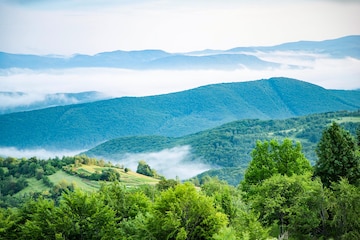This captivating image depicts a serene and lush forest landscape set against a sweeping mountain range. In the foreground, a dense array of tall, green trees covers the bottom half, offering varying shades of green—from dark to light. This rich forest scene seems to lead into a valley surrounded by rolling, tree-covered hills that stretch towards the horizon. Among the trees, there's a clearing on the hillside at the bottom left, framed by concentric rings of greenery descending into the valley on the right. The mountainous background appears bluish and extends from the left to the right edge of the image, partially obscured by clouds that settle among the peaks and valleys, giving an impression of floating mist. The sky above is predominantly white, streaked with clouds, suggesting an early morning setting as the sun begins to rise. This tranquil and picturesque scene evokes a tropical locale, possibly reminiscent of the Amazon rainforest or Hawaii.